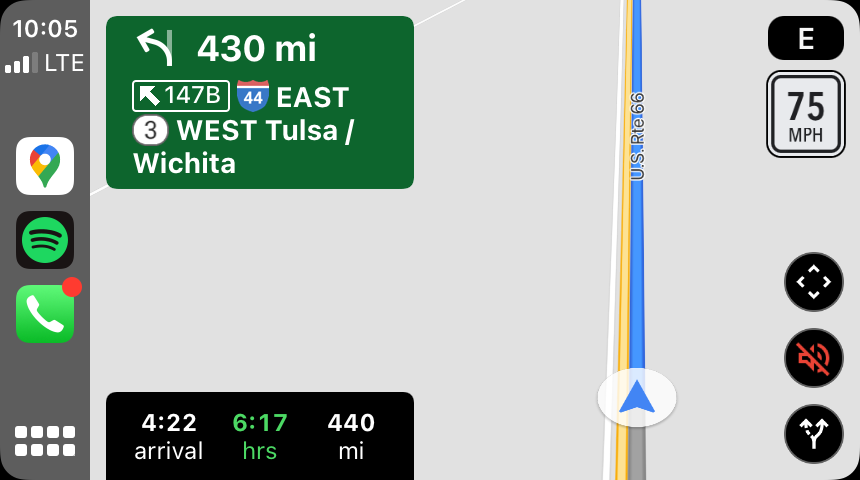**Detailed Caption:**

This image is a screenshot of a Google Maps navigation interface displayed on a smartphone in landscape mode. The phone's screen shows various interface elements and navigation details.

On the left-hand side, there is a gray navigation bar. At the top of this nav bar, the time is displayed as "10:05." Below the time, the cell signal strength is indicated with three out of four bars, accompanied by the "LTE" label. Further down, three app icons are visible: the Google Maps icon, the Spotify icon, and the phone icon, the latter marked with a red dot indicating a notification. At the bottom of this gray bar, there are eight small white squares arranged in a 4x2 grid.

The main part of the screen is the map itself. The map background is predominantly gray, indicating the navigational route and surrounding areas. The route being followed is highlighted in blue and marked as US Route 66. The traffic flowing in the opposite direction is denoted by a yellow line. 

In the upper-right corner, within a black rounded rectangle, there is a white "E" symbol. Directly below this, the speed limit is displayed as "75 mph" on a sign shaped like a traditional street sign. Beneath the speed limit sign, there is a circular icon featuring four corners of a square, rotated to appear as a diamond shape. Hidden slightly behind these icons, there is a red mute icon. A little lower, another black circle contains two arrows: one solid arrow pointing in one direction and a dotted line pointing in the opposite direction.

On the left side of the map, adjacent to the navigation bar, a green box with rounded corners provides the next navigation instruction. This green box displays an arrow pointed slightly to the left along with the distance "430 MI." Below this, within a rectangle featuring an arrow, the text "147B" is displayed outside the rectangle. To the right of this rectangle is an Interstate sign labeled "44," followed by "EAST" in all capital letters. Further information includes a circle with the number "3" inside it, accompanied by the text "West Tulsa / Wichita."

Overall, the image provides a detailed and comprehensive view of the navigation route and essential driving directions.